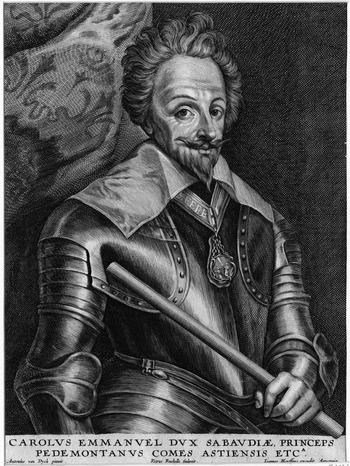The image is a detailed, hand-drawn black and white depiction of a distinguished and senior knight or nobleman. The artwork, characterized by meticulous shading, shows the man in profile, facing left. He is adorned in intricate metal armor, possibly from the 15th century, with visible plates over his chest and arms. Underneath the armor, he wears a long-sleeve undershirt with a collar. The knight's adornments include a noteworthy medal or medallion that hangs from a ribbon around his neck, bearing a crest at the center of his chest, likely indicating a station of high rank or honor.

His facial features are distinctive, with a pointed goatee that extends to his chin and a handlebar mustache that curves upwards. He has large, expressive eyes and a notably large forehead. In his left hand, he holds a slim rod or stick which rests diagonally across his chest.

The background is predominantly dark, with a shaded black area and a hint of a tapestry on the left side. At the bottom of the image, there is a legend written in non-English text, possibly Spanish, reading: "Calvary's Immanuel D.V.X. Sabavidel, Princeps Primontavs Cum Aesthetis E.T.C." This text adds an air of mystery and historical context to the image. Overall, the artwork appears to be more of a pencil or painting sketch, with a somewhat cartoonish style rather than photorealistic.